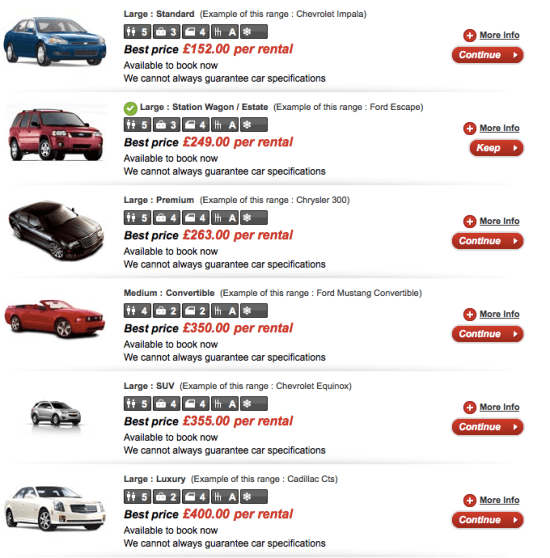The image depicts a page from a car rental service with a clean white background. On the left side of the page, there are six images of different vehicles arranged vertically. From the top, the vehicles are a blue sedan, a red SUV, a black sports car, a red convertible, a silver SUV, and a white Cadillac or luxury vehicle. 

In the center of the page, the rental prices for these vehicles are displayed. The pricing starts at $152 per rental for the blue sedan, followed by $249 per rental for the red SUV, $263 per rental for the black sports car, $350 per rental for the red convertible, $355 per rental for the silver SUV, and $400 per rental for the white Cadillac or luxury vehicle.

On the far right, there are interactive buttons designed to help users get more information and proceed with the rental process. Each vehicle listing includes a plus sign with a "More Info" label, indicating a clickable section for additional details. Below each "More Info" section, there is a prominent red button with white letters that says "Continue," inviting users to proceed to the next step in the rental process.